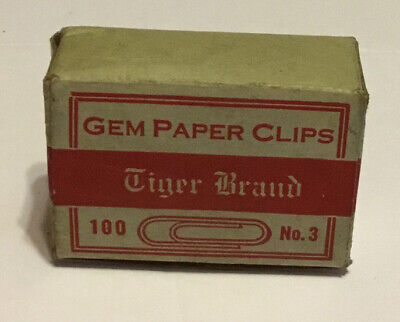The image depicts a vintage, worn cardboard box of Jim Paper Clips. The rectangular box is primarily a beige or grayish-tan color with various dents and beat-up spots indicative of its age. The front of the box features red text at the top declaring "Jim Paper Clips," followed by a wide red stripe, or band, with "Tiger Brand" printed in white letters. Below this stripe, on the left side, the number "100" is displayed in red, denoting the quantity of paper clips inside. Adjacent to this, there is an illustration of a paper clip, and to the right of it, the text "Number 3" specifies the size of the paper clips. The entire box rests on a beige or very light blue background, further highlighting its nostalgic appearance.